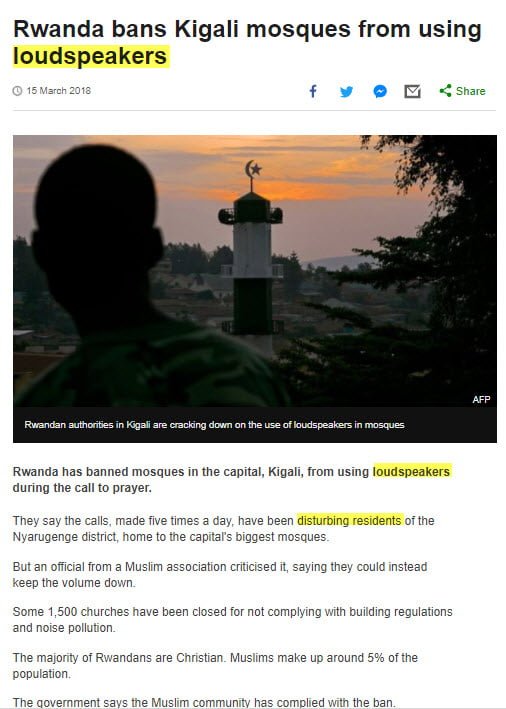Photograph capturing the exterior of the Kigali Mosque in Rwanda, dated March 15, 2018. The image reflects the controversy following Rwandan authorities' crackdown on the use of loudspeakers in mosques, specifically during the call to prayer. Highlighted in the photo is an instance of this regulation being enforced in the Nyarugenge district, home to Kigali's largest mosque. A man is seen standing outside the mosque, illustrating the human element of this policy's impact. The authorities have argued that the five daily calls to prayer, broadcasted via loudspeakers, have been disturbing to local residents. An official from a Muslim association criticized the ban, suggesting that a reduction in volume would be a better alternative. This event occurs within the larger context of Rwanda closing approximately 1,500 churches for non-compliance with building and noise regulations, in a predominantly Christian nation.